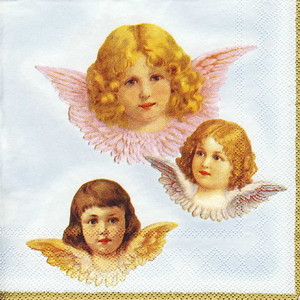The image is a detailed painted portrait of three young angels, capturing only their heads and the wings extending from their shoulders, set against a light blue and white, possibly hazy gray, background. The top angel dominates the upper section of the image. She has curly blonde hair, blue eyes, pink lips, and pink wings, conveying a serene expression. To her bottom right is a second angel with darker, curly hair and light bluish wings. The third angel, positioned slightly to the left of the center at the bottom, has brown hair that curls inward at the ends and yellow wings. Each angel's youthful and angelic faces, reminiscent of children around seven or eight years old, contribute to the ethereal and enchanting quality of the artwork.